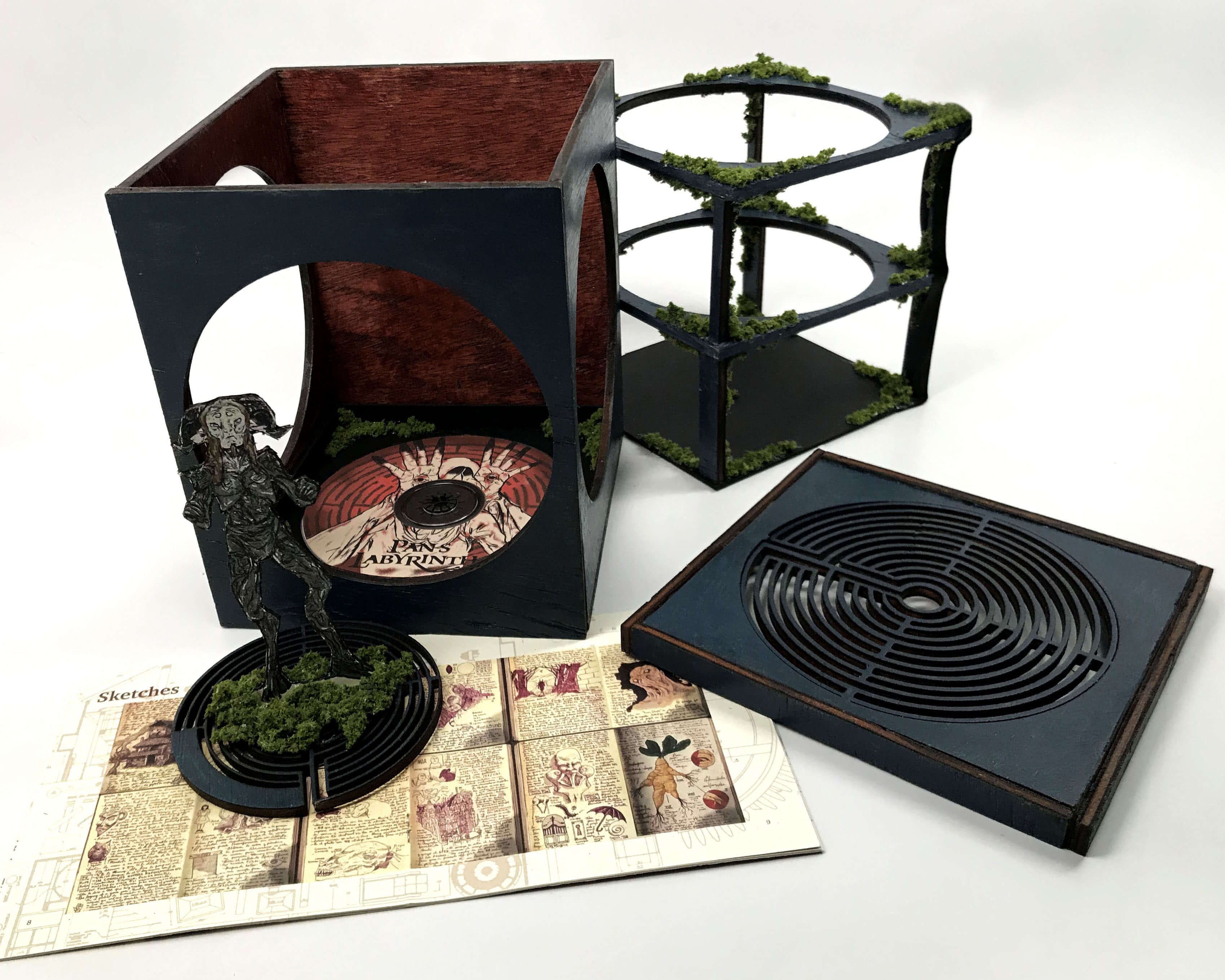This photograph shows an intricate collection of items against a flat white background. Central to the image is a black wooden box with three large circular cutouts on the front, left, and right sides, exposing its intricately detailed interior. Inside, the box is lined with rich, cherry wood. The box contains a creature-like model standing on a round platform, which is positioned on what appears to be green moss. This detailed figure, often described with goat-like features and outstretched hands, stands on a concentric circular pattern resembling those found in a Zen garden.

Adjacent to the box, there is a three-tiered structure with large circular holes in each tier, also adorned with moss. This structure closely fits inside the box and appears to be designed to hold and display the creature model. The lid of this box, which is possibly resting beside or underneath it, has similar concentric circles on it, suggesting a coherent design intended to house and view the statue even when the box is closed.

Also visible in the image are additional items, including a CD with an intricate design, and a comic book styled sketch art laid flat beneath some of the other components. The collective arrangement emphasizes a dark, mysterious theme, accentuated by the black exterior and rich wooden interior of the box, the eerie statue, and the detailed environmental elements like the moss and circular patterns.